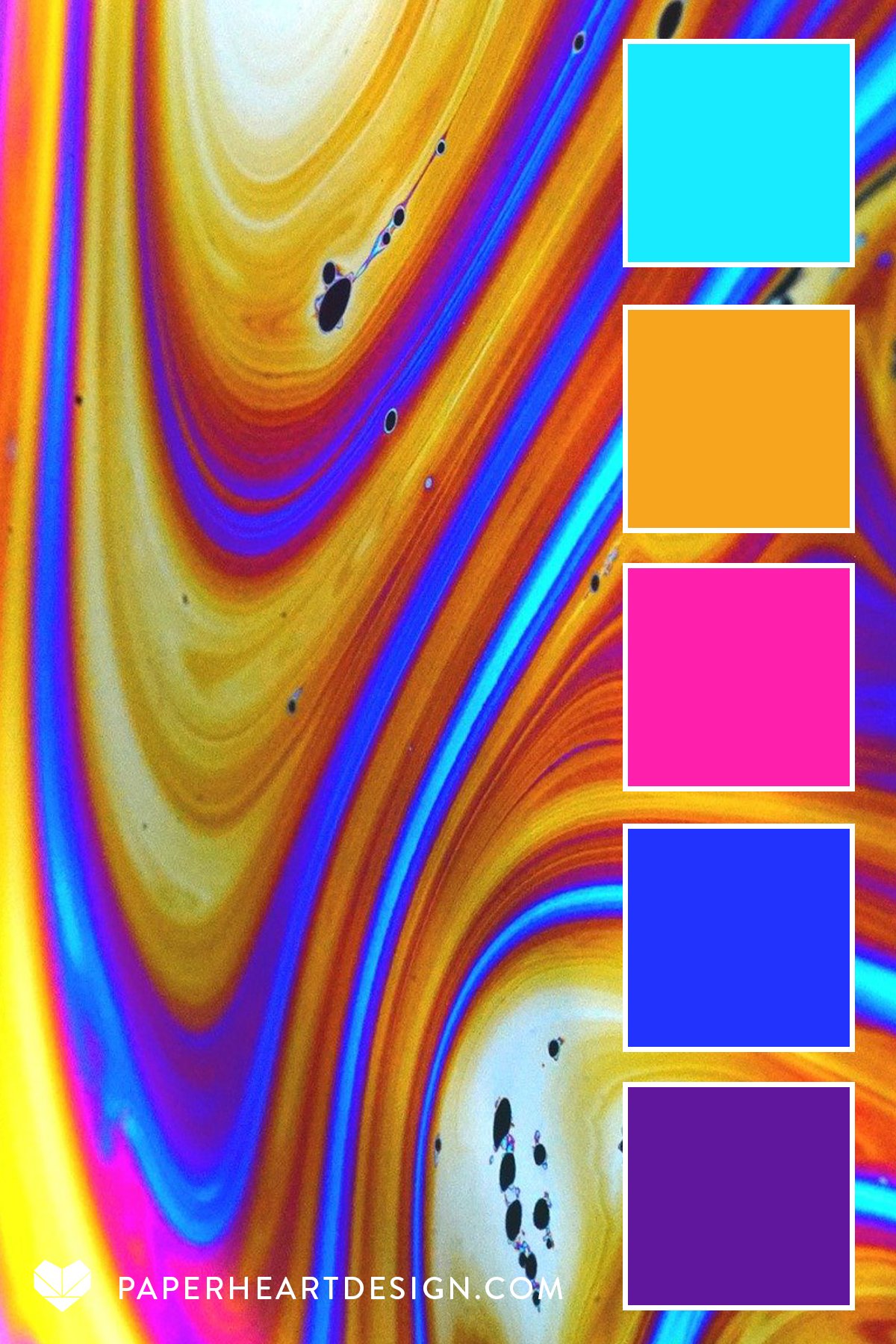The advertisement image is an abstract, vibrant, and visually striking piece of modern art. Dominated by swirling patterns and neon hues, the image radiates outward from a central, sun-like yellow circle at the top. The swirls transition through a spectrum of colors: yellow, red, purple, darker green, gold, pink, and bright blue, interspersed with areas of orange and black dots.

On the right side of the image, there is a vertical column of five colored squares, each showcasing the primary colors found within the artwork. From top to bottom, these squares are light teal, orange, magenta, dark blue, and purple. These colors reiterate the composition’s vibrant palette.

Additional details include fluid, fluorescent rings reminiscent of planetary bands and abstract liquid swirls. Notably, in the lower-left corner of the image, the modern art piece is branded with "paperheartdesigns.com" in white capital letters, combining elegance with a commercial touch.